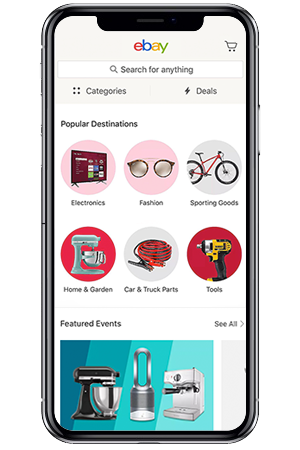In the image, there is a gray cell phone displaying an eBay webpage. At the top of the screen, the eBay logo is prominently featured with its distinctive red "e," blue "b," yellow "a," and green "y." Below the logo, there is a shopping cart icon and a search bar that reads "Search for anything," accompanied by a magnifying glass icon.

Further down, a grid labeled "Categories and Lightning Deals" is showcased. Beneath this, the section heading "Popular Destinations" appears, followed by icons and images representing various categories:
- **Electronics**: Depicted here is a large flat-screen TV.
- **Fashion**: Illustrated by a pair of glasses.
- **Sporting Goods**: Represented by a bright red 10-speed bicycle.
- **Home and Garden**: Shown with a gray stand mixer featuring a large silver bowl.
- **Car and Truck Parts**: Illustrated by a set of jumper cables.
- **Tools**: Represented by a power drill.

Under these categories, there is a section titled "Featured Events," accompanied by a "See All" link and a right-pointing arrow. 

This is followed by a highlighted blue box showcasing additional items: a black stand mixer with silver trim and a large silver bowl, an air diffuser, and a Keurig-type coffee machine.